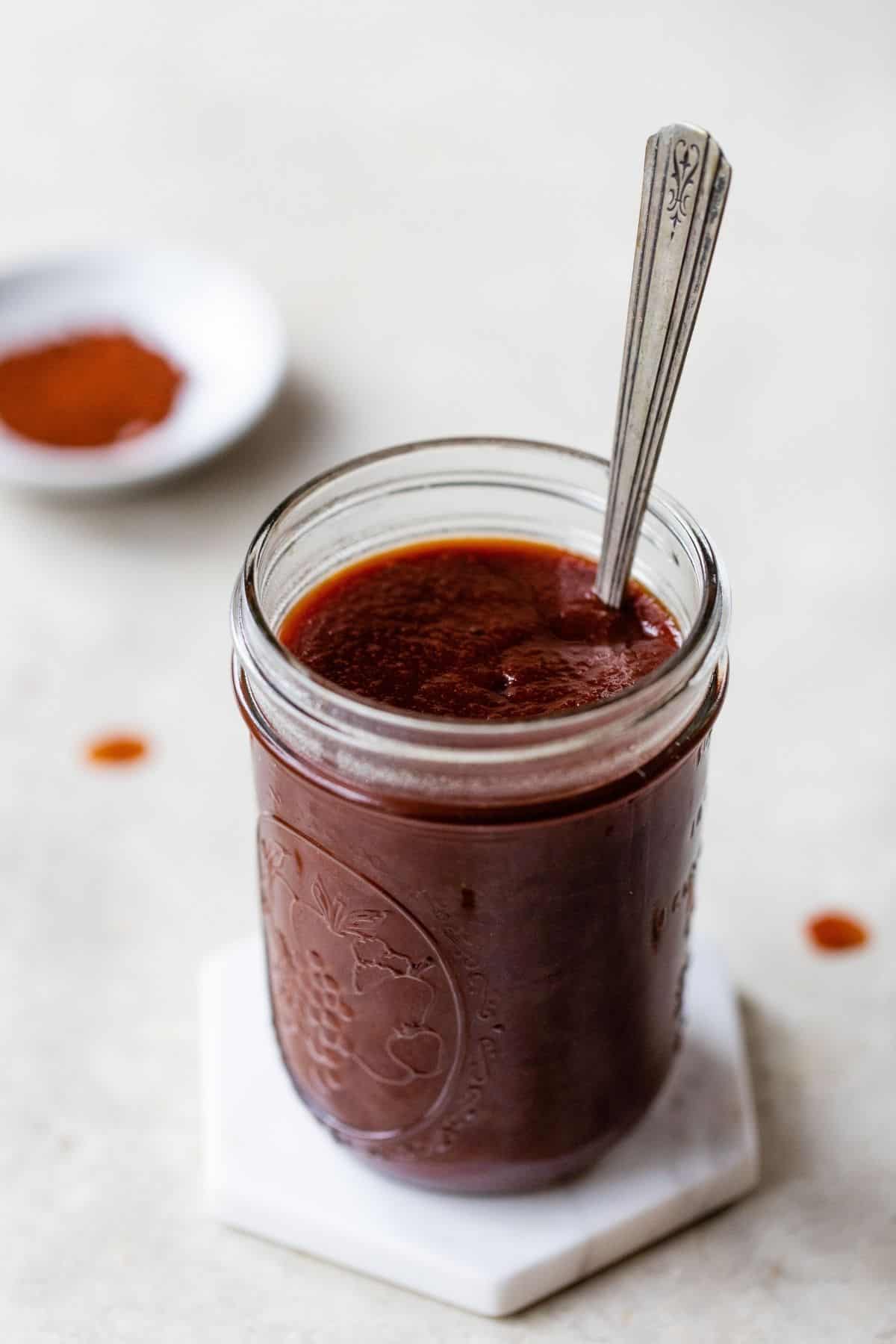The image presents a detailed and focused view of an open glass jar filled with strawberry jam. The jar, adorned with intricate engravings depicting various fruits such as grapes, apples, strawberries, and pears, stands elegantly on a hexagonal white marble coaster. A silver spoon is inserted upright into the thick, rich jam. Surrounding the jar, to the left and right, are a few drips of jam on the white surface, suggesting slight spillage. In the background, the top left features a blurred white plate or saucer containing a small amount of jam. The engraved fruits on the jar are in relief, adding a textured contrast to the clear glass, while the overall scene is meticulously captured with a shallow depth of field, highlighting the jar of jam as the central focus.